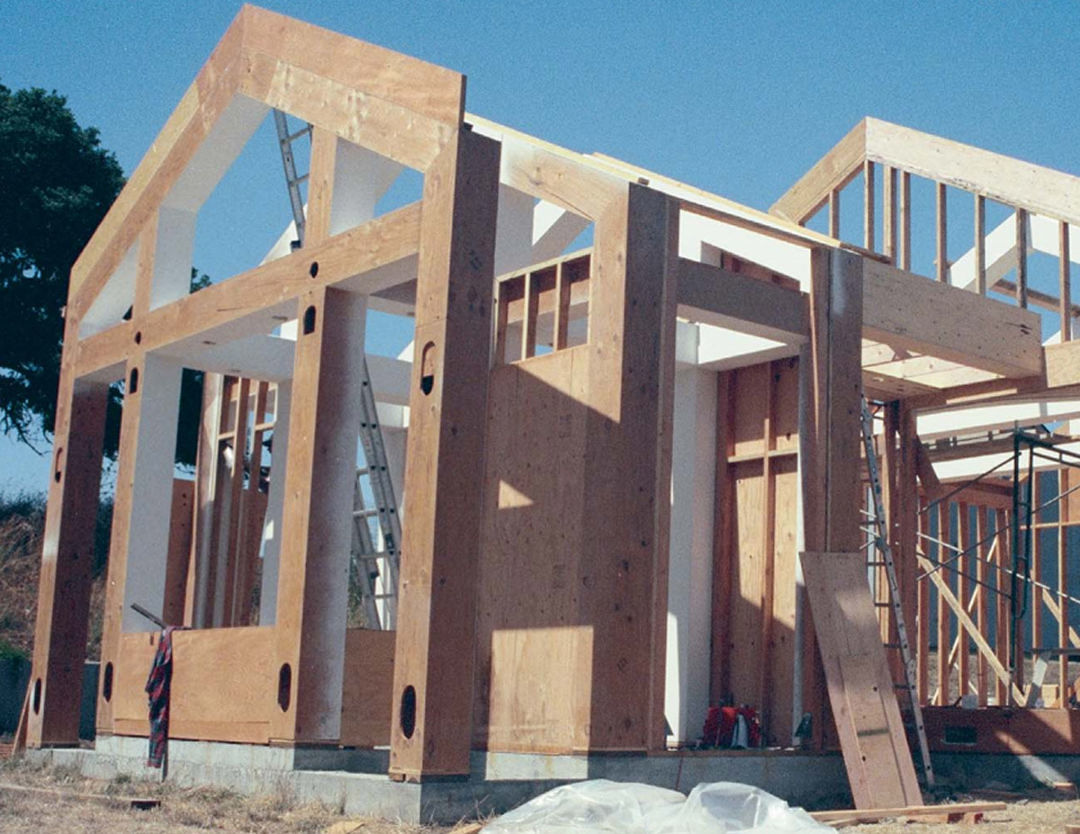The image captures an outdoor setting under a clear, blue sky devoid of clouds. Dominating the left side of the frame is a tall, lush green tree. The centerpiece of the photograph is a wooden structure in the midst of construction, which could potentially be a house or a church, noted by its peaked front and dual doorway design. The wooden frame is diligently set up, with ladders strategically placed throughout the interior, including one extending from the floor to the roof behind the door frame. The construction site features various scattered elements: several plastic bags lie around the dirt-covered ground, a red and blue plaid button-down shirt dangles off the frame of the door, and unassembled planks of wood are strewn about next to the cement foundation. Additionally, there are distinct oval holes in the wood at the front of the structure, hinting at the architectural detailing in progress.